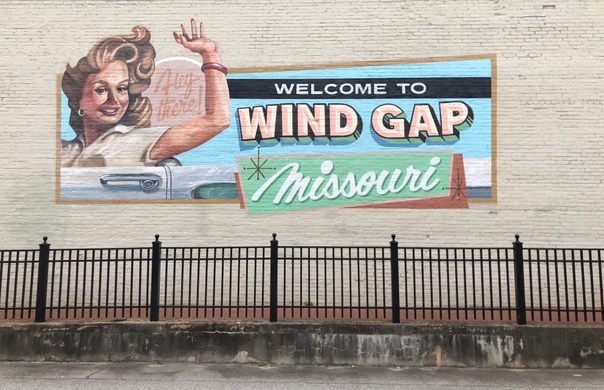The image is a vibrant and detailed depiction of a vintage advertisement painted on the side of a cream-colored brick building. The ad features a cheerful 1950s-style scene with a smiling, wind-blown blonde woman waving energetically from a silver convertible car. She is dressed in a white, retro blouse and wearing gold or silver earrings, capturing the essence of mid-century charm. Prominently displayed in light blue, pink, and green lettering is the welcoming message, “Welcome to Wind Gap, Missouri,” with “Welcome to” in black font. The phrase “Hey there” appears near the woman's arm, enhancing the friendly and nostalgic vibe. Below the painting, there is a walkway bordered by a black iron fence, and in front of that, a gray, slightly dirty sidewalk. The overall ambiance is bright and inviting, reflecting a sunny daytime scene that warmly invites viewers to the quaint town.